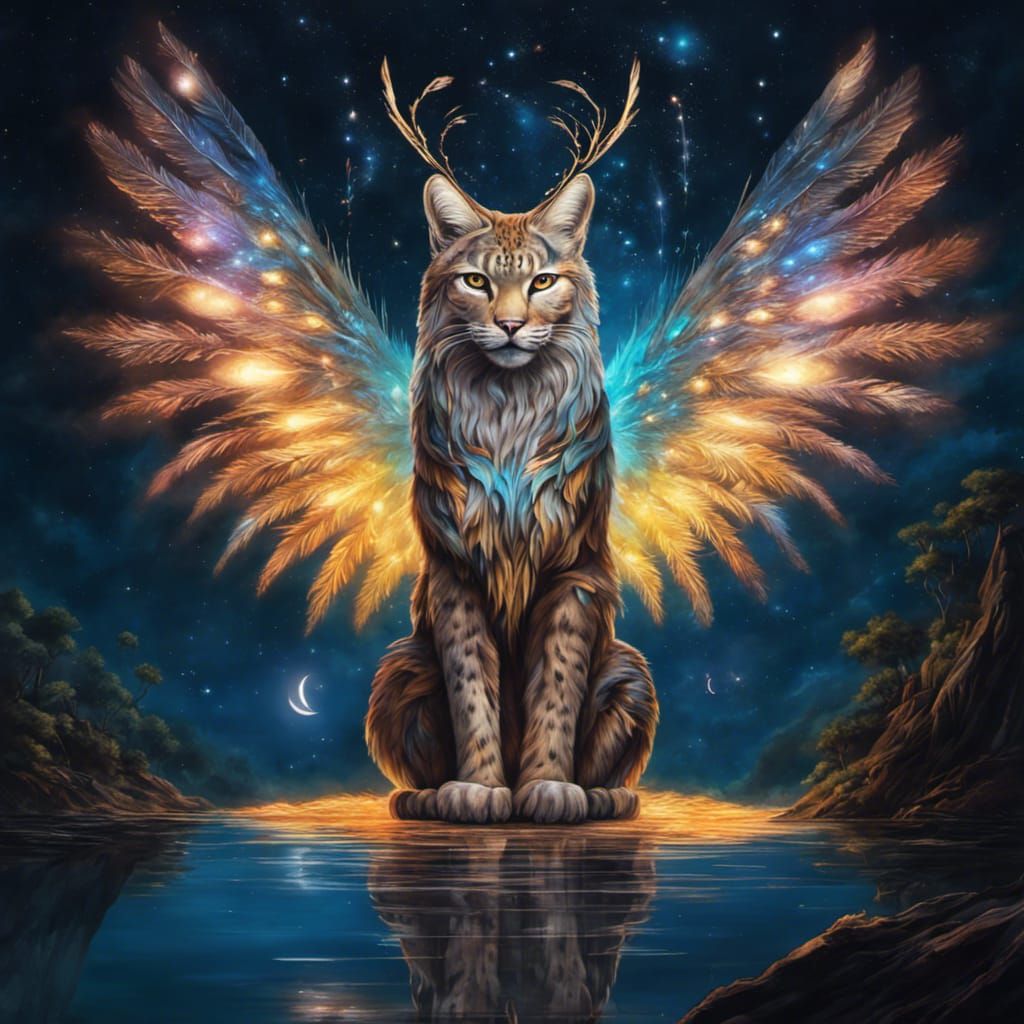This detailed fantasy-themed, computer-generated illustration features a majestic, twilight-lit scene with a unique, winged cat as the focal point. The cat, resembling a house cat with elements of a wild cat and the spotted markings of a leopard, sits serenely on a mirror-like pond surrounded by cliffs and trees. Its visage includes typical feline characteristics: whiskers, ears, and a normal house cat face, but also boasts a big, bushy white mane and curious features resembling twine-like horns. The feathery wings extending from its back are adorned with a myriad of illuminated colors—predominantly blue with pink and purple hues closer to its body, transitioning to an orange glow at the feather tips. Overhead, a dark blue, star-speckled sky and a radiant blue moon contribute to the ethereal ambiance, with sparkles accentuating the cat’s feathered wings and creating a celestial spectacle. The entire scene is reflected perfectly in the calm waters below, capturing the mystical essence of this enchanting digital artwork.